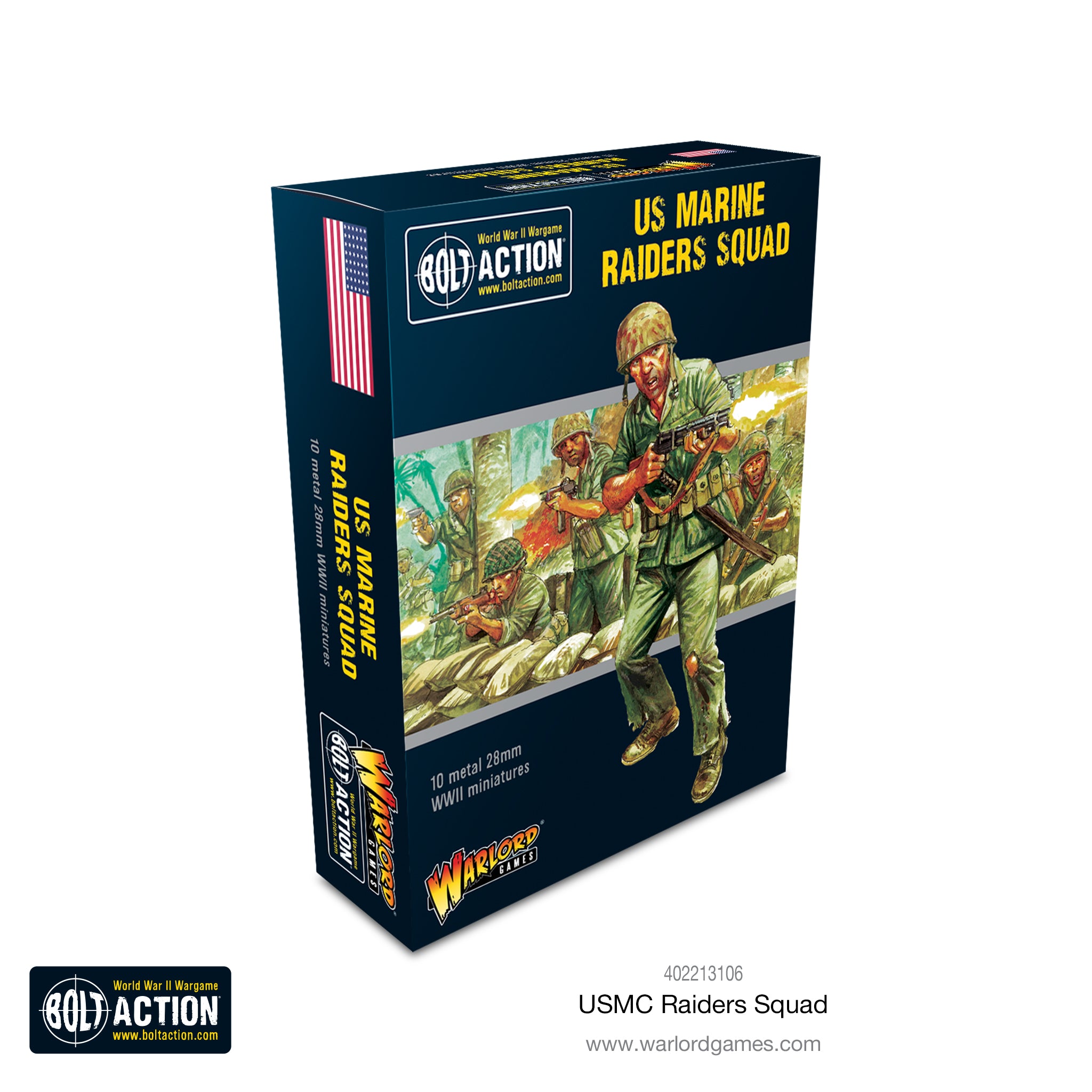The image depicts a predominantly black game box with detailed thematic artwork and informative labels indicative of a World War II miniature set. The most prominent feature at the top is the title "USMC Raider Squad" displayed in bold, yellow, all-capital letters against a black background. Below, the artwork illustrates American marines in olive drab uniforms, equipped with helmets and rifles, one of which appears to be firing, as indicated by the visible muzzle flash. The scene is set against a backdrop of a World War II battlefield, with additional soldiers positioned behind white sandbags. 

In the top left corner of the box, an American flag is visible, signifying the national identity of the depicted soldiers. Along the bottom of the illustration, descriptive text reads "10 Metal, 28mm, World War II Miniatures". The bottom also features a detailed annotation with the bold "Bolt Action" logo on the bottom left combined with the "Warlord Games" logo on the bottom right, adjacent to the website link: www.warlordgames.com. The number code 402213106 runs along the bottom edge, marking this specific product. The box uses a blend of military greens, yellows, and oranges to highlight the wartime theme, against its predominantly black background which enhances the vivid colors and detailed illustrations on the box.